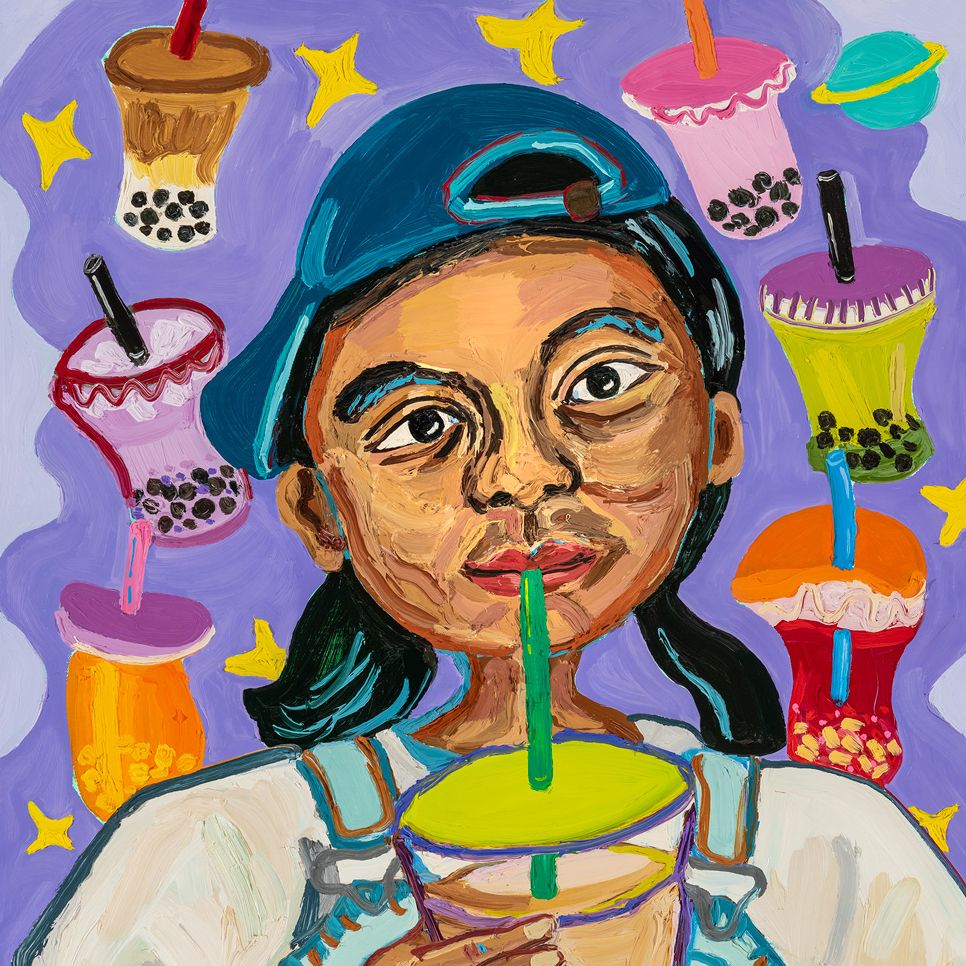The image is a vibrant and colorful painting of a stylized girl with a light brown complexion. She is depicted with black hair styled into two ponytails and wears a blue backwards cap. Her outfit consists of blue overalls with a white shirt underneath. The girl has a very round face with rosy lips and is drinking from a cup through a vibrant green straw, with the cup featuring a bright green lid and containing a beige-colored drink, reminiscent of bubble tea. The background is dominated by a purple hue adorned with various star and planet shapes, including a prominent teal-colored planet with a yellow ring in the upper right corner. Arranged behind the girl are six multicolored takeout-style cups, three on each side, each containing what appears to be bubble tea with distinctive tapioca pearls at the bottom, enhancing the whimsical and playful atmosphere of the painting.